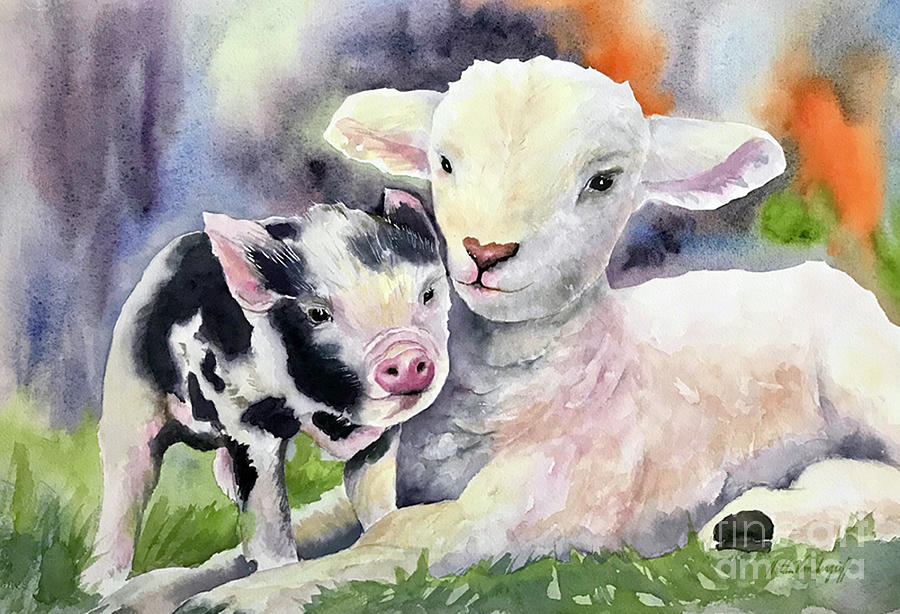This detailed watercolor painting, presented by Fine Art America, captures a tender moment between a baby lamb and a piglet. The lamb, perfectly white with a soft face, black hooves, and black eyes highlighted with a white dot, is lying on its stomach with its front legs outstretched and one hind leg visible. Its pink-nosed, fluffy ears are straight out with a pink underside. Nestled close to the lamb is a black and white piglet, primarily white but adorned with black spots on its face, body, and ears. The piglet stands on all fours, its pink snout and the insides of its ears adding a splash of color as it cuddles close, front legs straddling the lamb's limbs. Both animals gaze directly towards the viewer, exuding a sense of intimate companionship. The background features a serene watercolor blend of orange, light blue, purple, green, and hints of black and white, representing a stylized sky and ground. Different shades of green suggest a grassy setting at the bottom, framing this heartwarming pastoral scene. Faintly visible in the lower right corner is the text, "Fine Art America," marking the artwork's origin.